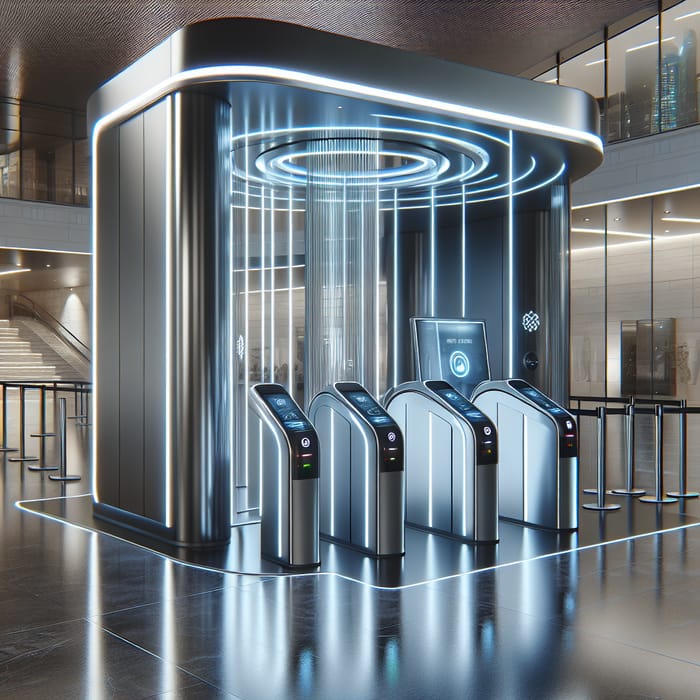The image shows a futuristic, automated security kiosk situated in a metallic and brightly lit indoor space. The focal point is a large central machine with a cylindrical compartment that extends vertically, surrounded by circular elements and white segments at the top. In front of this central unit, there are four distinct entry points resembling turnstiles, each equipped with keypads or small control panels. The area is cordoned off along the sides and back, with a shiny tiled floor that reflects the glow of the machinery. In the background, a staircase—possibly made of marble—leads to a second floor with railings overlooking the scene. On the right side, large windows offer a view of an exterior cityscape. The overall aesthetic is sleek and modern, reminiscent of an airport security checkpoint, with a sign providing operational instructions, though the text is not legible.